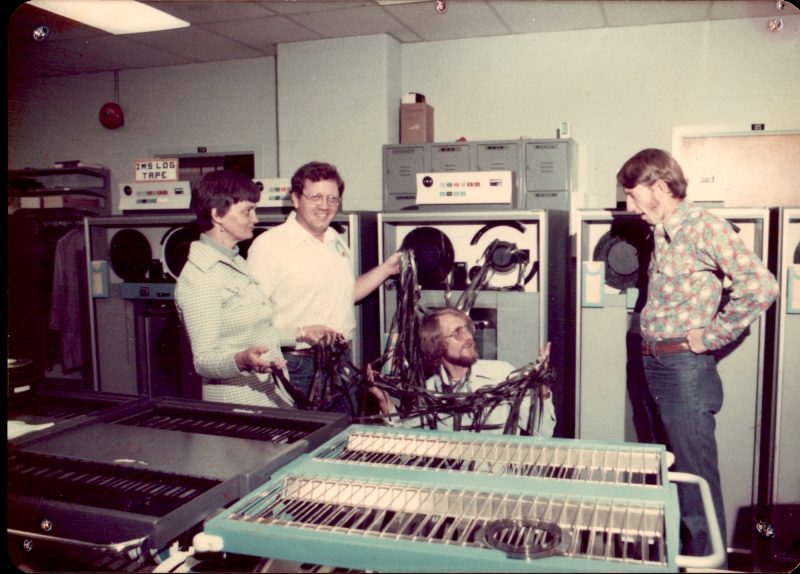In this vintage photograph from the mid to late 1970s or early 1980s, a group of four individuals is gathered in a light-gray room with lowered ceilings and a fluorescent light fixture in the upper left-hand corner. The room, likely a recording or radio room, is equipped with bulky, old-style tape decks against the walls. The focal point of the image shows one woman and three men standing in a loose circle. The woman, dressed in a light blue turtleneck and a checkered suit, gazes towards the man to her right. This man is looking down at another man seated on the floor, who is gazing up at him. All three are holding torn strands of audio tape, creating a jumbled mess. Another man stands to the right of them, hands on his hips, seemingly caught in mid-sentence as he surveys the scene. The background is filled with large tape machines, enhancing the nostalgic feel of the photo with metallic grates and reels. The attire, complete with loud shirts, pinstripe suits, and era-specific hairstyles and accessories, firmly roots the image in its time period.